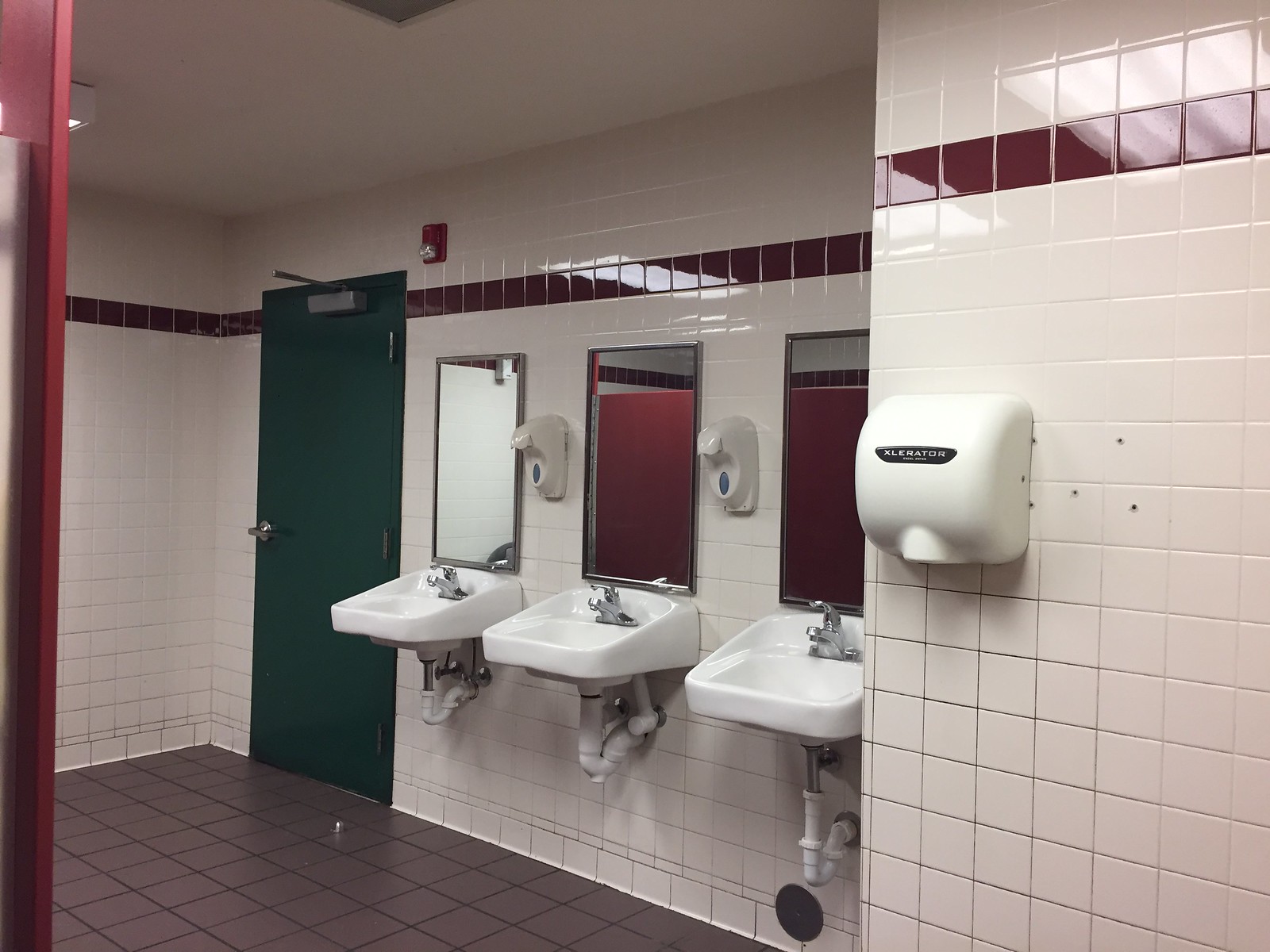This image depicts a commercial bathroom characterized by its clean, structured design. The walls are adorned with white subway tiles, punctuated by a dark maroon stripe located four tiles down from the ceiling that matches the color of the stall doors visible in the mirrors. The floor is covered in maroon tiles. The right side of the bathroom features a green exit door, next to which sits a fire alarm. Adjacent to this, three white porcelain sinks are mounted below three separate mirrors, with two soap dispensers positioned between the mirrors. A commercial hand dryer is installed on the right wall, completing the functional layout of this well-maintained bathroom space.